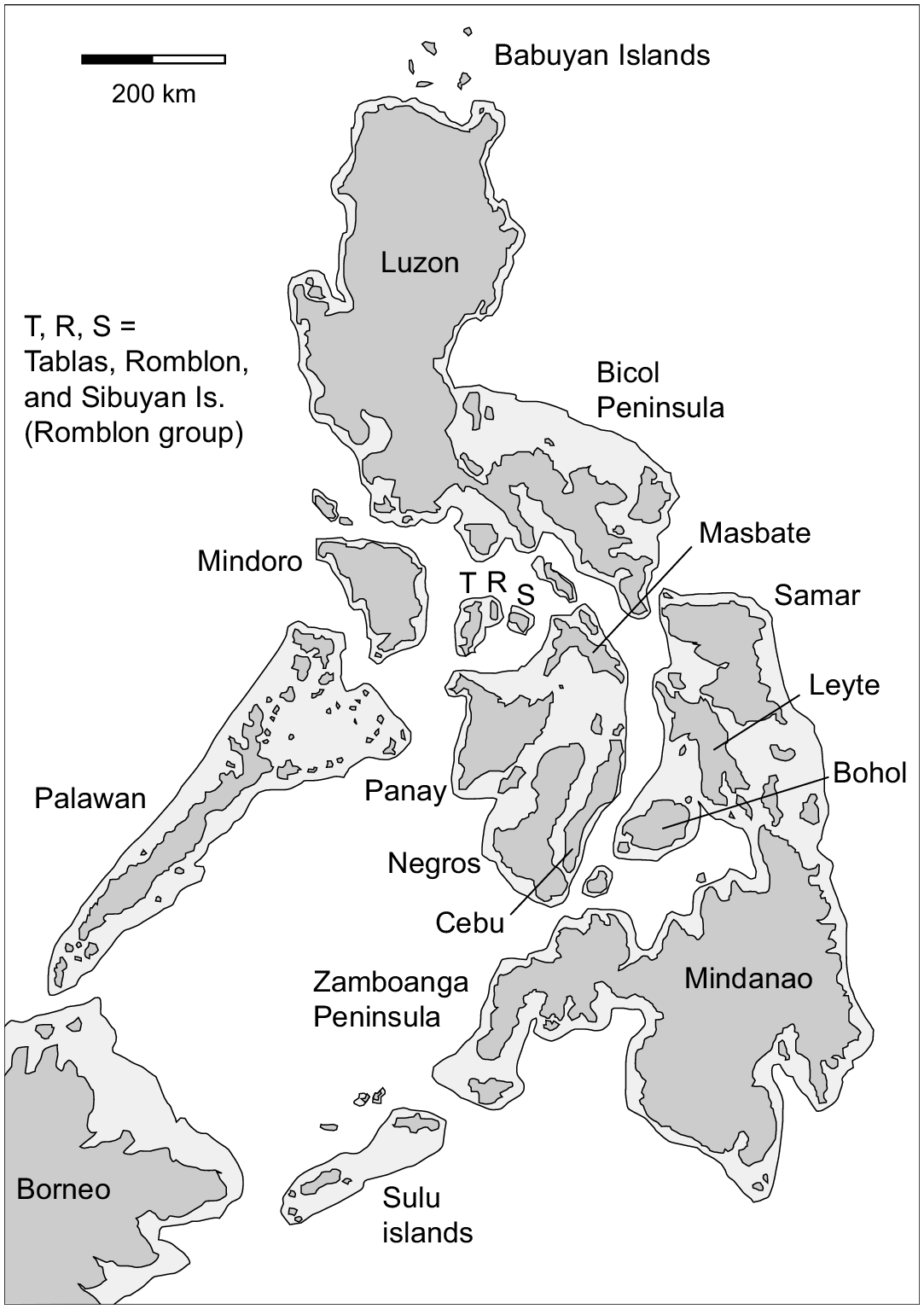The black and white map prominently features an archipelago stretching from the top right to the bottom, with several islands extending to the left. In the top left corner, a black and white bar indicates a scale of 200 kilometers. Each island is shaded in dark gray, outlined by a lighter gray, with the surrounding background in white.

At the top center of the map, the Ababayan Islands are labeled. Below this, the large island of Luzon is situated, followed by the Bicol Peninsula. Beneath the Bicol Peninsula, three islands are collectively labeled as T-R-S (Tablas, Romblon, and Sibuyan Islands), known as the Romblon group.

To the left of these, the larger island of Mindoro is marked. Further down to the left, the long, narrow island of Palawan stretches out. To the right of Palawan, a sequence of islands is identified: Masbate at the top, followed by Panay to the lower left, Negros directly below, and Cebu to the right of Negros.

Further to the right, another group of islands is denoted; Samar is at the top, Leyte below it, and Bohol to the lower left of Leyte. The large island of Mindanao is situated further down, with the Zamboanga Peninsula extending to its left. Beneath Mindanao, the Sulu Islands are labeled, consisting of two larger islands and several smaller ones. In the bottom left corner, part of the landmass is labeled as Borneo.

Each island label is written in black text, ensuring clarity against the shades of gray. The map's legend explains the abbreviations T-R-S as Tablas, Romblon, and Sibuyan Islands, referred to collectively as the Romblon group.